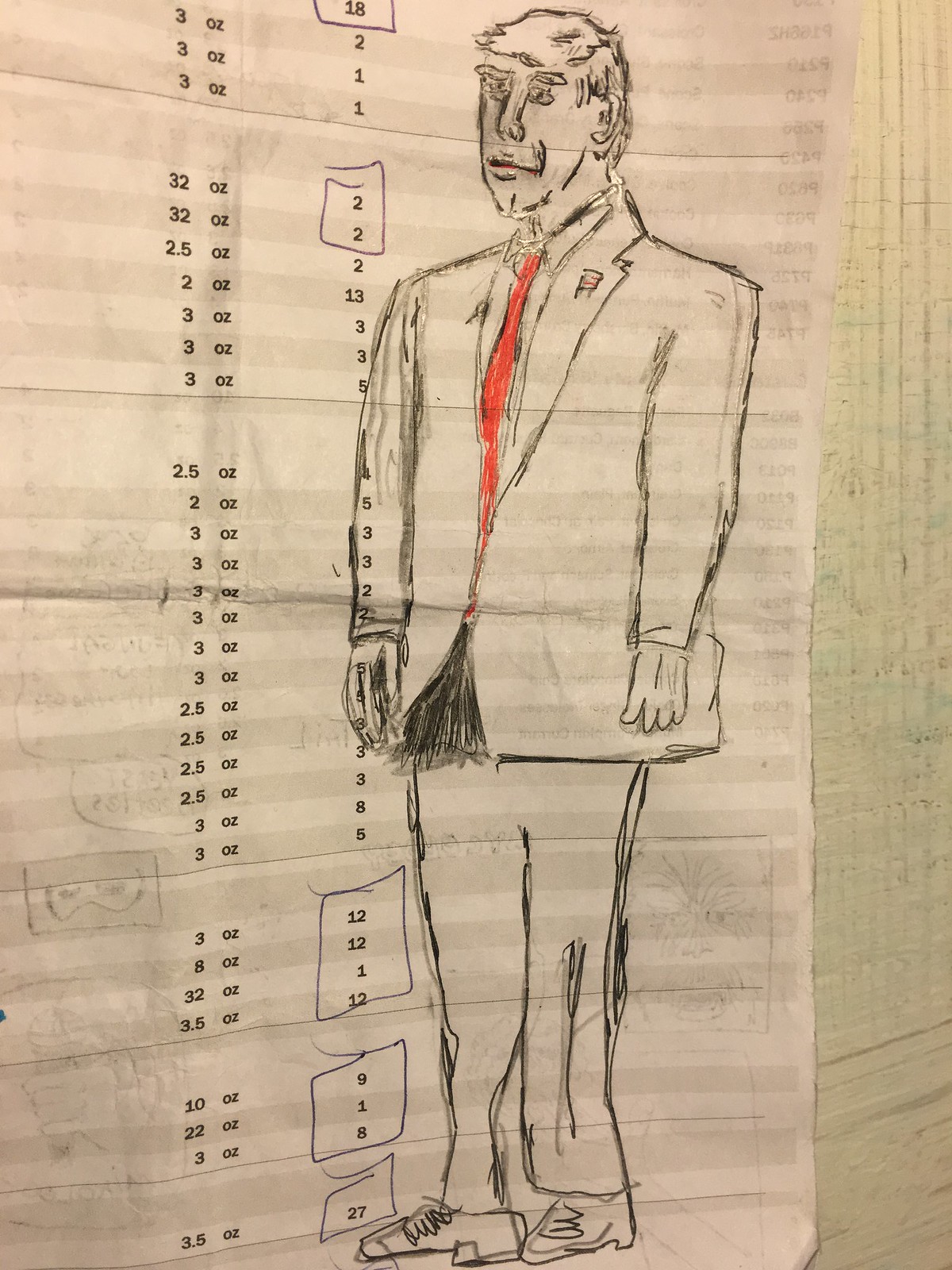The image on the screen is a detailed black-and-white pen drawing of a man in a suit, who closely resembles Donald Trump. The only color in the artwork is found in his tie and a small lapel pin, both exhibiting a reddish-orange hue. The man is depicted in a partial side view, facing left and looking off-screen. The figure stands with arms at his sides, showcasing four discernible fingers on his left hand, while the right hand's fingers appear less defined due to shading. He wears a buttoned-down shirt that is fastened up to his chin beneath the suit.

The man has a clean-shaven face, with only his eyebrows adding a touch of hair to his visage. His hair is neatly parted to the right, extending just below his ears. Broad shoulders and an imposing height give him a commanding presence, a likely intention of the artist.

Alongside the figure, there are two vertical columns of measurements. The first column, situated from above the man's head to his feet, lists approximately three dozen incremental measurements ranging from 3 ounces to 32 ounces. The second column features numeric values starting from 18, occasionally boxed off, descending to 2, including an isolated 27 amidst the sequence. These details collectively contribute to the structured and meticulous nature of the composition.